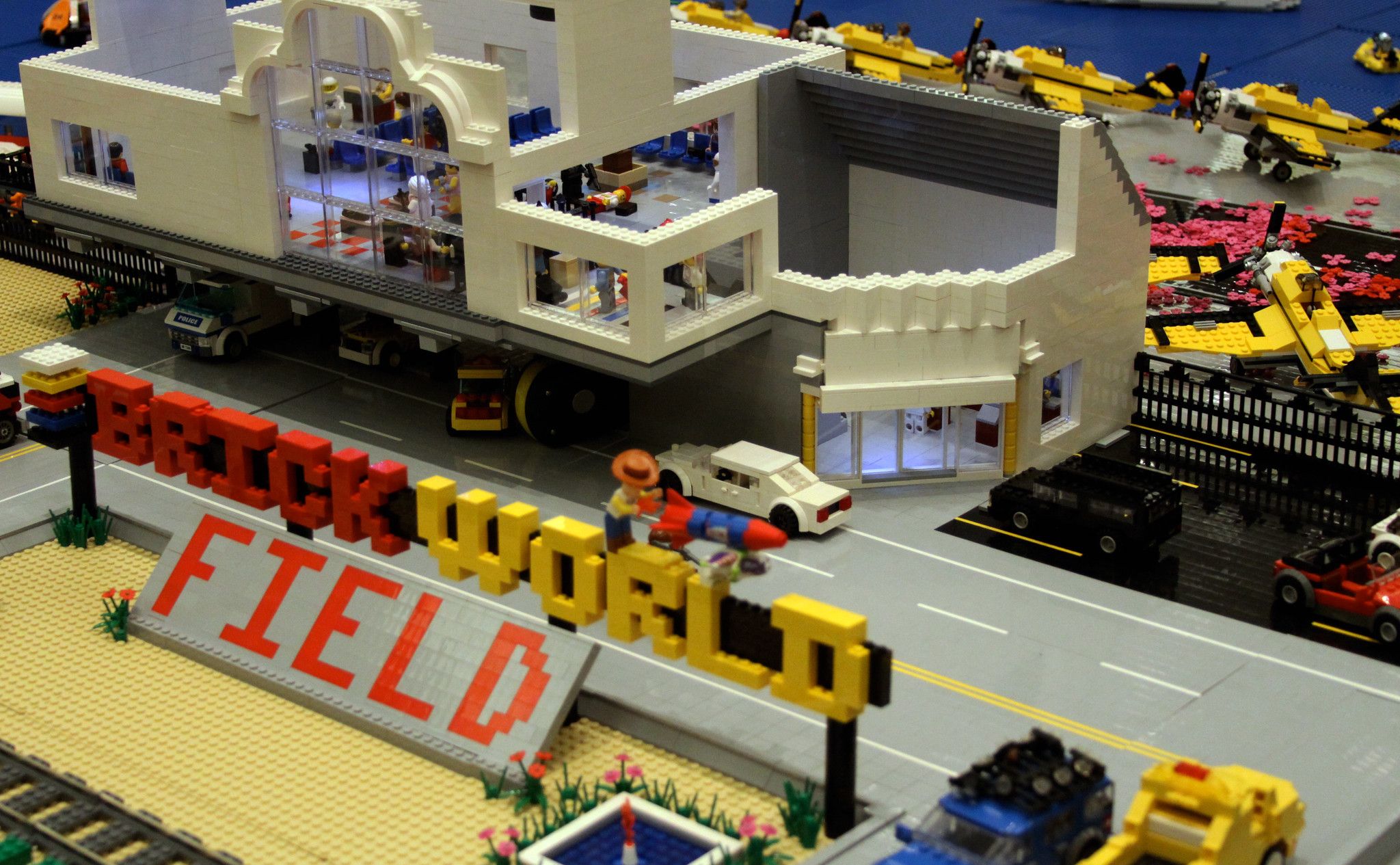This highly detailed photograph captures an intricate Lego construction scene centered around a diagonal street. On the right-hand side, there is an open-air building resembling an airplane hangar. This structure lacks a roof and reveals a collection of small yellow planes—four to five in total—parked within the space. Adjacent to this hangar, atop a white platform with red and white checkered flooring and an archway with windows, are various toy brick figures that appear to be pilots.

On the left side of the street, labeled "Brick World Field" with "Brick" in orange, "World" in yellow, and "Field" in red or orange lettering on a gray background, lies a beige-colored field. This field features scattered flowers and a small water area. Nearby, there are a few automobiles: a blue car, a yellow car, and a white car. Additionally, a toy figure holding a red rocket stands prominently atop the "Brick World Field" sign.

Further details include extra toy figures and trucks scattered throughout the scene, adding layers to this detailed miniature representation. The overall construction supplies a vibrant and bustling microcosm, rich with activity and meticulously crafted elements.